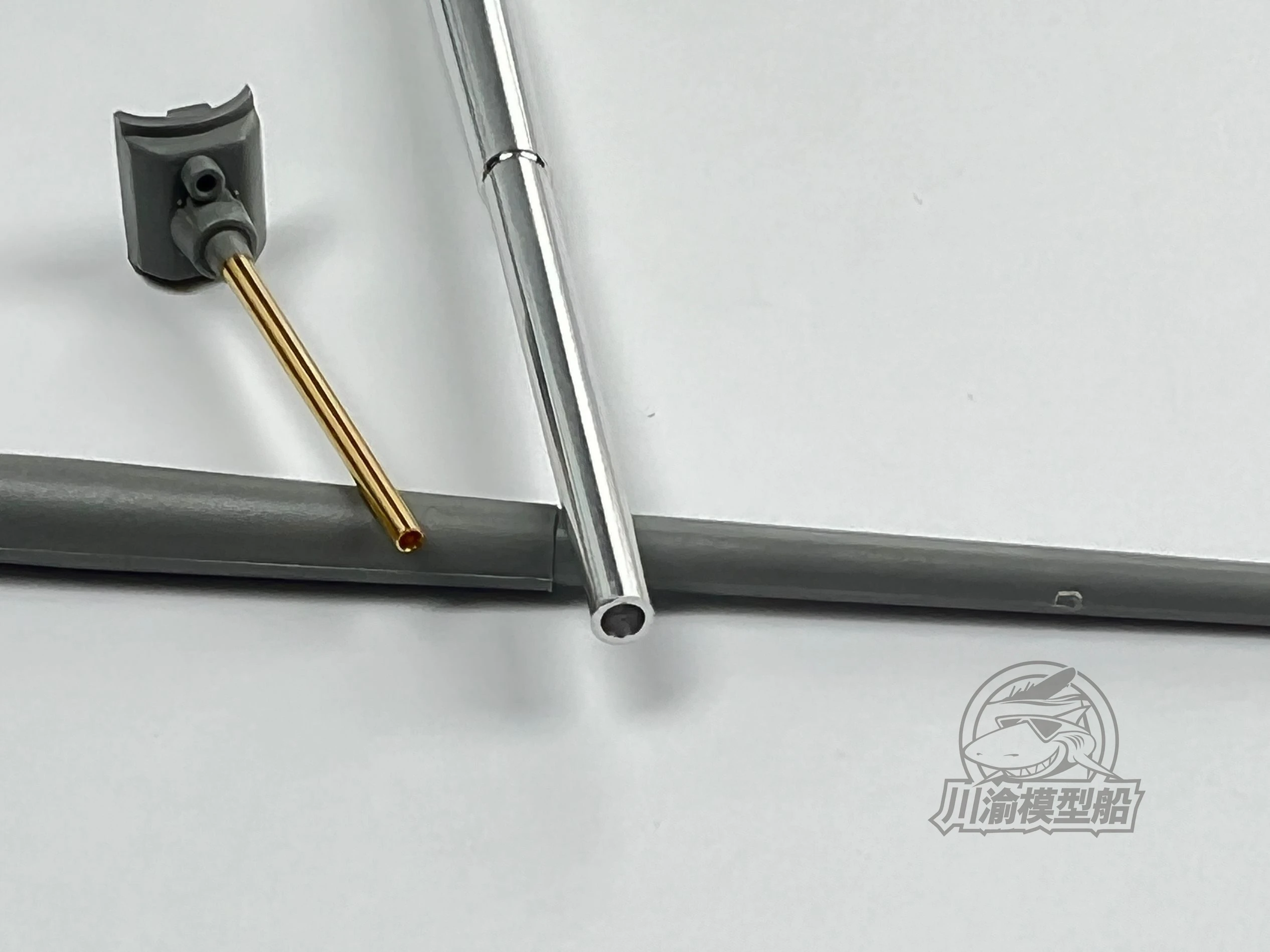The image features three distinct tubular objects arranged on a grayish-white gradient background. Each object appears unique and seems to serve a different purpose. The first object is a brass rod connected to a plastic component, resembling a handle; it has a circular metal piece projecting a few inches from its top. The second object is a silver rod made of brushed chrome or stainless steel, and it appears to be telescoping, with two sections that fold into each other. The third object is made of dark gray plastic and is laid beneath the other two, also having a telescopic design. All three rods look somewhat like pens owing to their cylindrical shapes.

In the bottom right corner of the image, there is a logo featuring a smiling cartoon shark adorned with sunglasses, facing towards the left, and seemingly wearing a feathered accessory. Below the shark, there are Japanese characters. The background of the image adds a professional, understated backdrop to the eclectic assortment of objects.